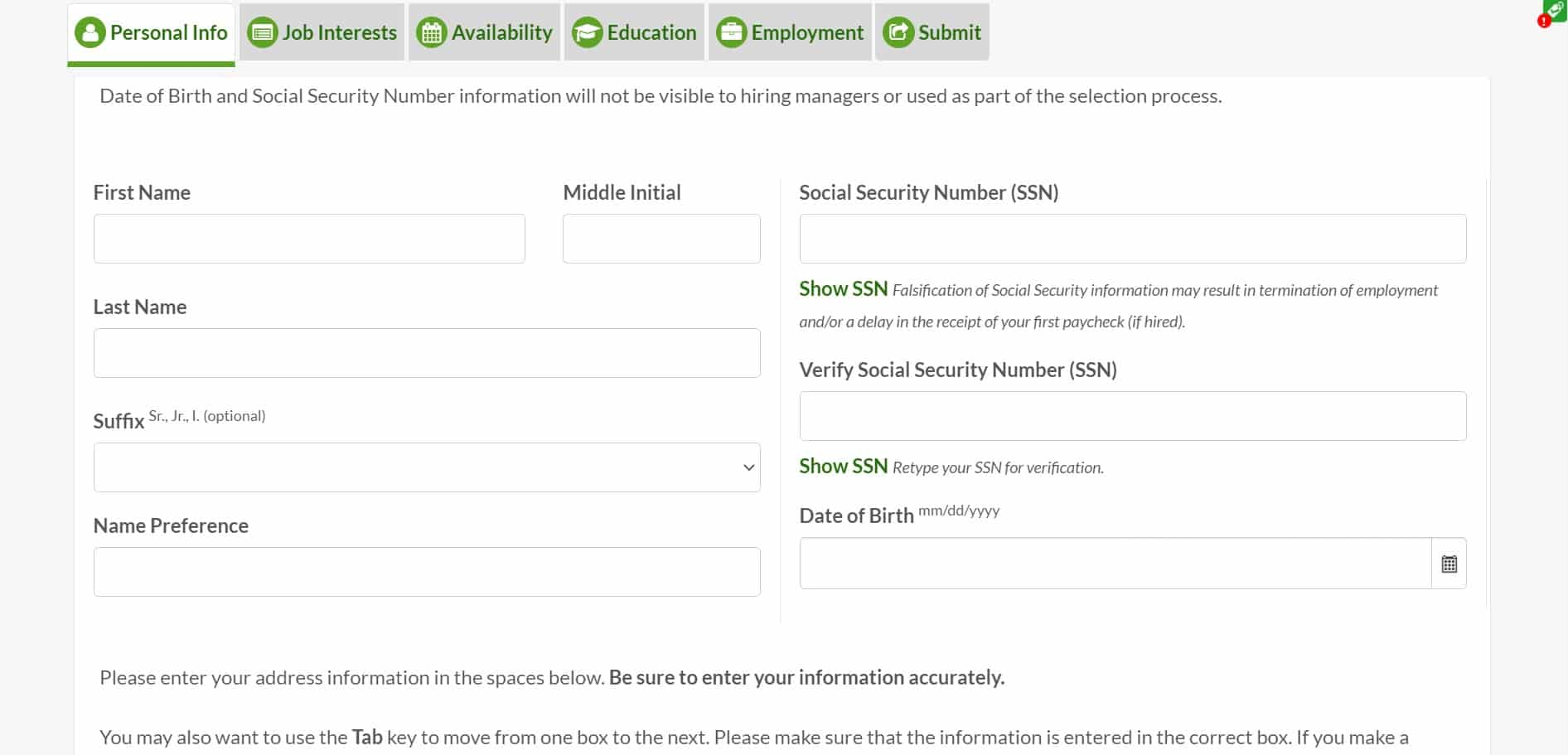The webpage displayed features a predominantly white color scheme with a very pale grey background. At the top of the page, there is a navigation bar consisting of six tabs oriented from left to right. 

1. **Personal Info:** The tab is highlighted in green, with a circular icon depicting a white head and shoulders silhouette.
2. **Job Interests:** This tab has a green circular icon containing a white symbol next to the label.
3. **Availability:** It features a calendar icon in white set against a green background.
4. **Education:** The icon shows a graduation cap within a green circle.
5. **Employment:** This tab displays an office building icon in white within a green circle.
6. **Submit:** The icon is a white symbol within a green circle.

In the upper right corner, there is a small green square with a red dot. 

Currently, the “Personal Info” tab is active, distinguished by its white background. At the top of this section, there is a notice in tiny font stating, "Date of Birth and Social Security Number information will not be visible to hiring managers or used as part of the selection process."

Below this notice, the form is divided into two columns:

**Left Column:**
- **First Name:** Label with a corresponding text box below it.
- **Middle Initial:** Label with a text box next to the First Name field.
- **Last Name:** Label with a text box beneath Middle Initial.
- **Suffix:** Label with a drop-down box option below Last Name.
- **Name Preference:** Label with a text box at the bottom of the left column.

**Right Column:**
- **Social Security Number (SSN):** Label with an option in green text to “Show SSN." There is a warning stating, "Reveal of Social Security Information may result in termination of employment and/or delay in the receipt of your final paycheck."
- **Verify Social Security Number (SSN):** Label with a text box to re-enter SSN.
- **Date of Birth:** Instructions to enter the DOB in "MM/DD/YYYY" format followed by a text box.

Further down the page, there is a broader section stating, “Please enter your address information in the spaces below. Be sure to enter your information accurately. You may also want to use the Tab key to move from one box to the next. Please make sure that the information entered is in the correct box. If you make a…” (the text is cut off here).

This thorough layout ensures users can systematically input their personal details while being guided through specific fields to fill out.